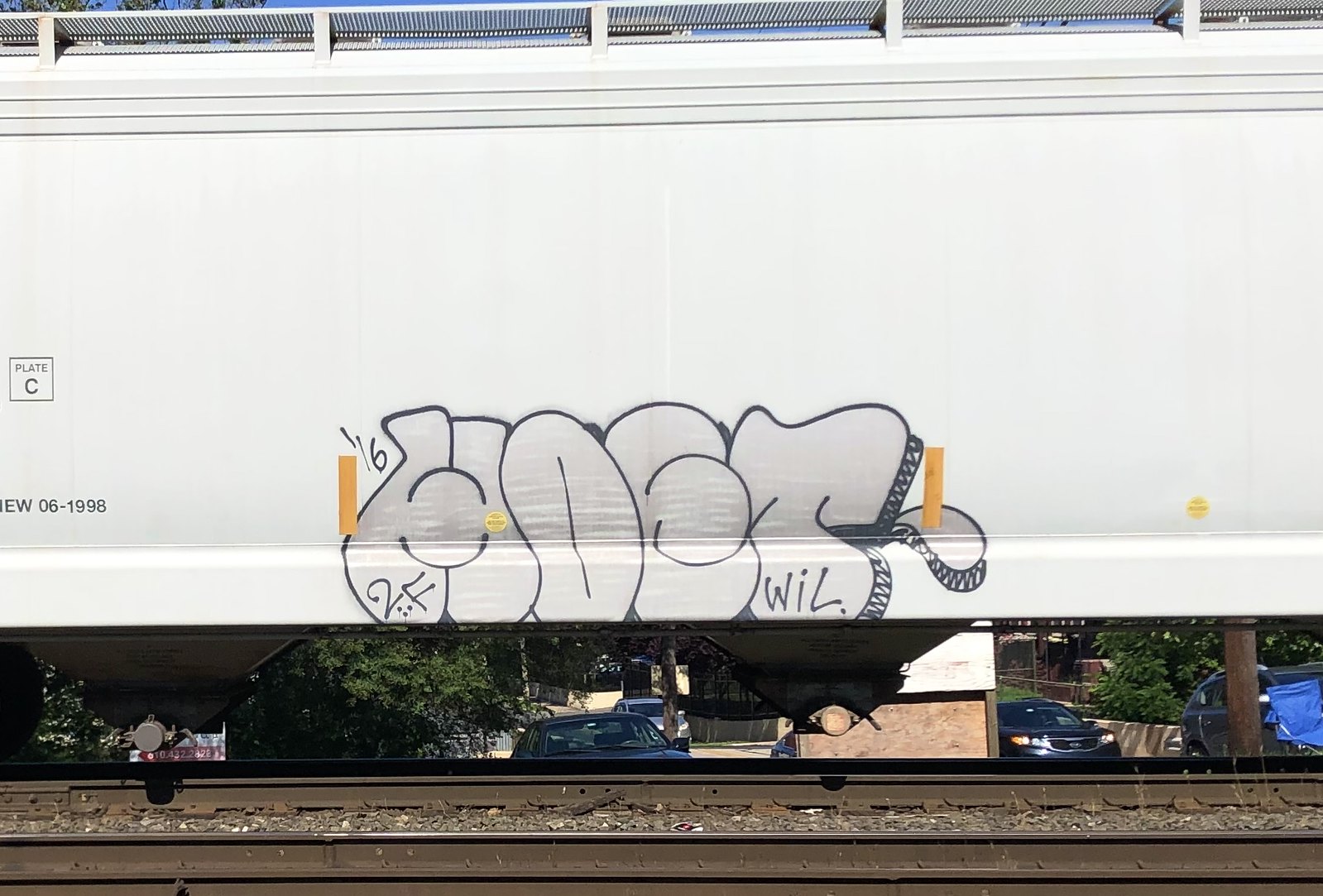The image captures a detailed scene of a white train car adorned with illegible graffiti, which appears to be a blend of interpretive artwork or bubble letters. The graffiti, centralized on the white surface, features large letters and includes elements such as "H-O-E-T" and the signature "W-I-L," along with two yellow plates on each side and a label stating “Plate C,” accompanied by the initials “E-W-O-6-1-9-9-8.” Below the train car, the brown, slightly rusted railroad tracks are visible, with the gravel and open space between the bottom of the train and the tracks allowing a view of multiple parked cars, buildings, and lush green trees in the background. The scene is captured during the daytime, with sunlight enhancing the details of the train and its surroundings.